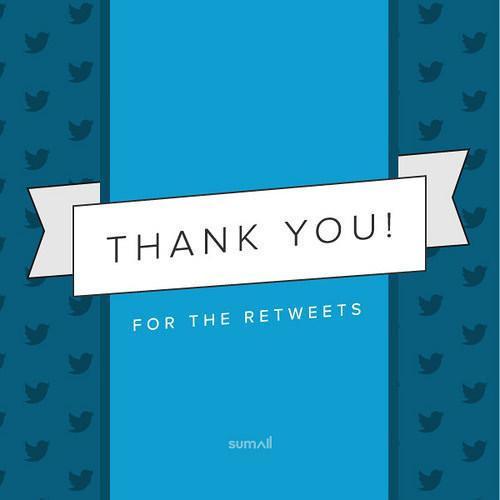The image appears to be an old Twitter-themed digital thank-you card. It features a horizontal white ribbon banner in the center set against a light blue background. This central banner prominently displays the text "Thank You!" in black font. Directly beneath this, the banner reads "for the retweets" in a smaller white font. Framing the light blue background are dark blue borders on the right and left sides, each adorned with multiple rows of dark blue Twitter bird emblems, depicting birds in flight. Below the "thank you" message, the text "sumall" is written in smaller white font on the light blue background, which may refer to the sender or recipient. Overall, it's a stylized and detailed Twitter graphic expressing gratitude for retweets.